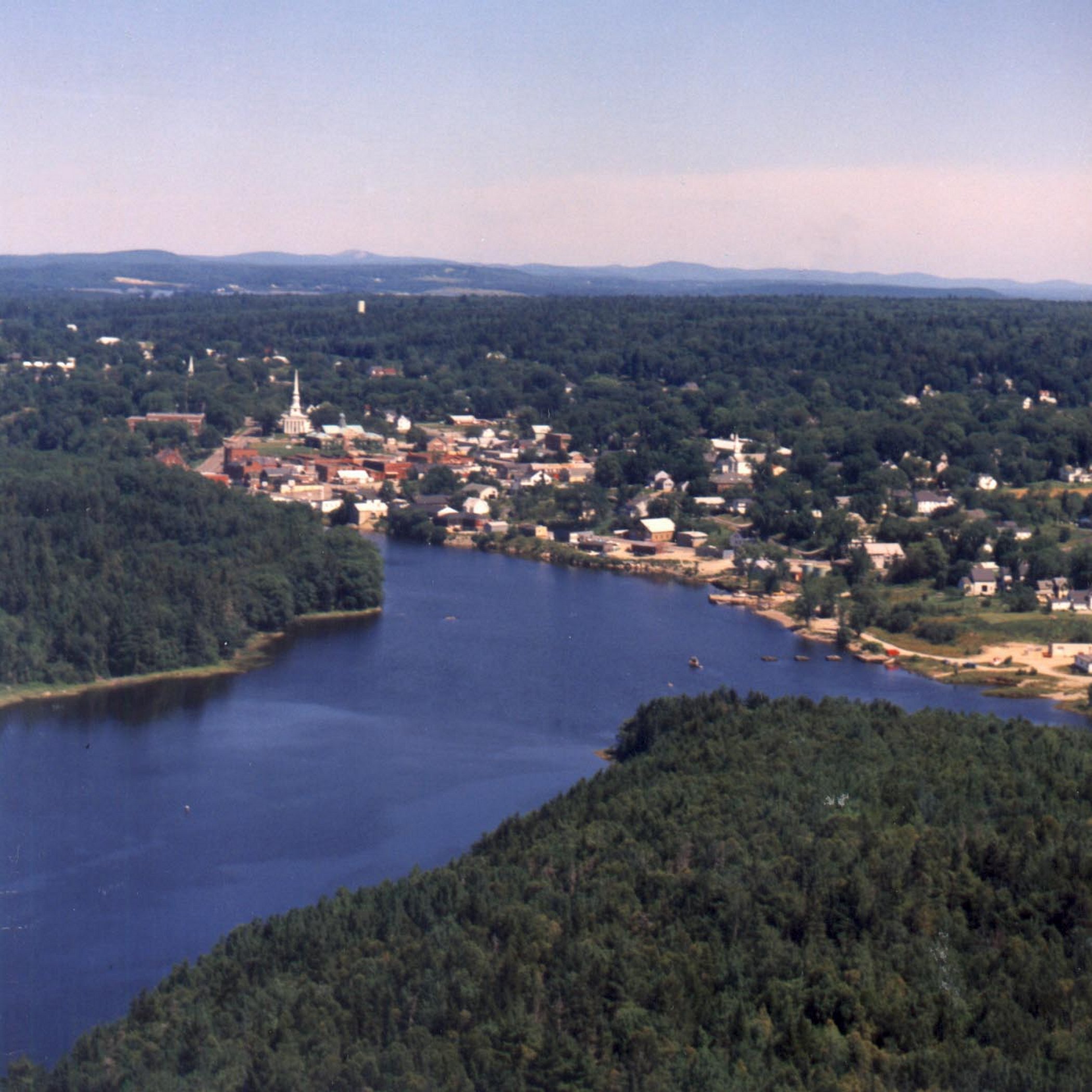This aerial photograph, though grainy and low in quality, captures a picturesque scene of a wide, serene lake flanked by dense forests and a quaint town. Starting from the bottom left and stretching towards the middle of the image, the lake is bordered on one side by an almost impenetrable mass of trees, their density allowing no glimpse of the ground below. To the right and above the lake lies a collection of buildings, predominantly brown with white roofs, nestled among yet more trees. The buildings become sparser as they stretch toward the right side of the image, suggesting a blend of urban and natural landscapes. In the upper left corner, a prominent church with a steeple stands tall among the other structures, indicating this area to be the heart of the town. Beyond the town, the vista opens to a distant horizon of rolling mountains under a mostly cloudy sky that graduates to a clear blue as it extends upward, encapsulating the tranquility and timeless charm of this serene, riverside town.